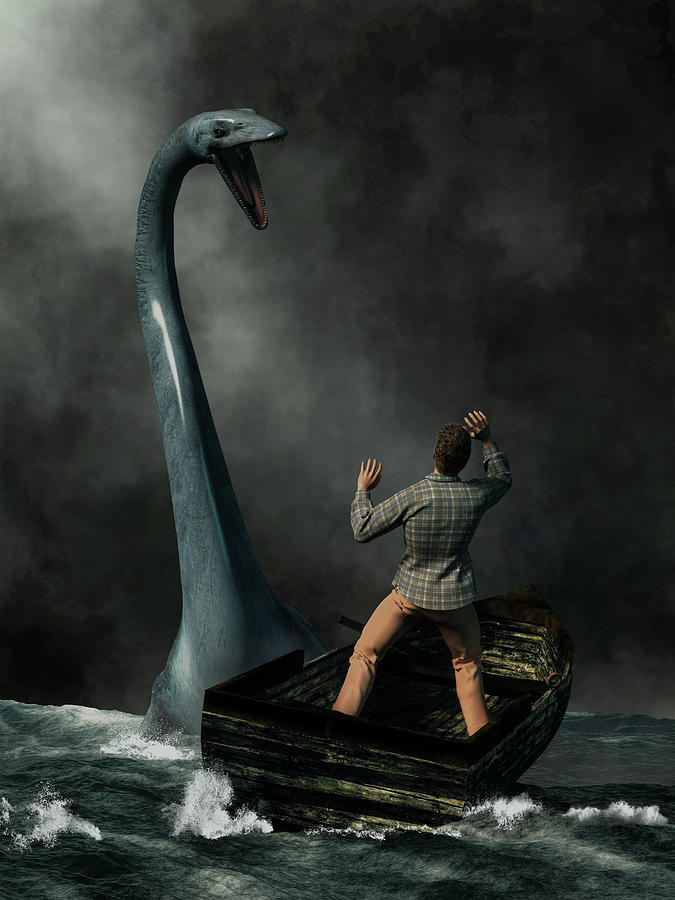In the image, a dramatic scene unfolds under a dark, stormy sky with shades of black and gray. The rough, churning water below showcases little crests of waves. A man stands in a small, weathered wooden canoe, which appears to be adrift without any paddles. He is viewed from the back, wearing an orange or khaki pair of pants and a checkered or plaid long-sleeve shirt, and has his arms raised, possibly in a defensive posture. His dark brown hair is noticeable. To his left, a giant, snake-like sea creature—colored in hues of gray-green with hints of blue—emerges from the water with its mouth wide open, exposing tiny sharp teeth. The creature, reminiscent of myths like the Loch Ness monster, appears menacing and possibly angry, adding an element of imminent danger and tension to the scene. The overall composition suggests a stylized or possibly staged scene rather than a natural occurrence.